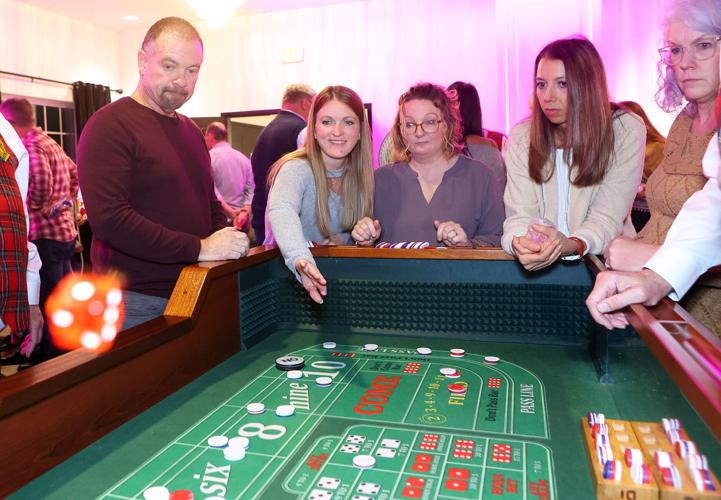In the center of the room, a lively casino scene unfolds around a green craps table. A group of five people—one man and four women—engage passionately in the game. The man stands to the left, identifiable by his short hair, beard, and mustache, dressed in an oxblood sweatshirt. Beside him, a younger woman with long, blond hair, clad in a blue top, is captured in the act of throwing orange dice with white dots. 

Adjacent to her stands an older woman with shorter, blond hair, wearing glasses and a v-neck gray top. Another young woman with longish brown hair, dressed in a white shirt and tan jacket, is nearby. On the far left, an older woman with short gray hair and glasses wears a brown vest. A glimpse of a dealer’s hand, emerging from a white shirt, hovers over the table.

Chips are scattered across the table, which is marked with essential game elements including the numbers "6" and "9," and sections labeled "COM," "PASS," and "RUN." The background reveals other patrons engaged in various activities at different booths, suggesting this might be a casino night event rather than a typical Las Vegas setting. The predominant colors in the scene range from greens and browns to occasional pops of red, set against pink-hued walls, adding to the vibrant atmosphere.